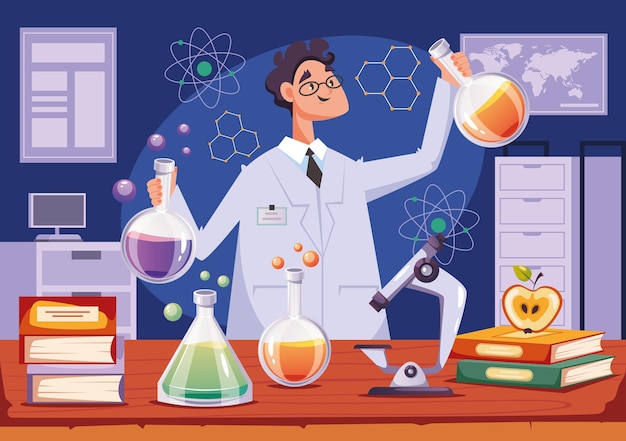This detailed digital graphic captures a scene of a scientist, likely a chemist, immersed in an experiment within his lab. The square, borderless image features a white male scientist with curly black hair, black glasses, a black tie, and a gray lab coat. He holds two round-bottom flasks in his hands—one containing an orange liquid and the other a purple liquid. 

On the desk in front of him, there are various scientific instruments and items: to the far left, a stack of three books or binders, a green beaker bubbling with substances, a gold beaker, a steel-colored microscope, and another stack of two notebooks. A halved apple rests atop the rightmost stack of notebooks. 

Behind the scientist, the wall is adorned with various molecule and compound drawings, adding to the busy, scientific atmosphere. A computer monitor is visible to the left, and a world map is positioned in the upper right corner, with a silver filing cabinet to its left. This vivid, multi-color digital artwork, reminiscent of illustrations found in children's scientific literature, brings the bustling energy of a chemist's lab to life.